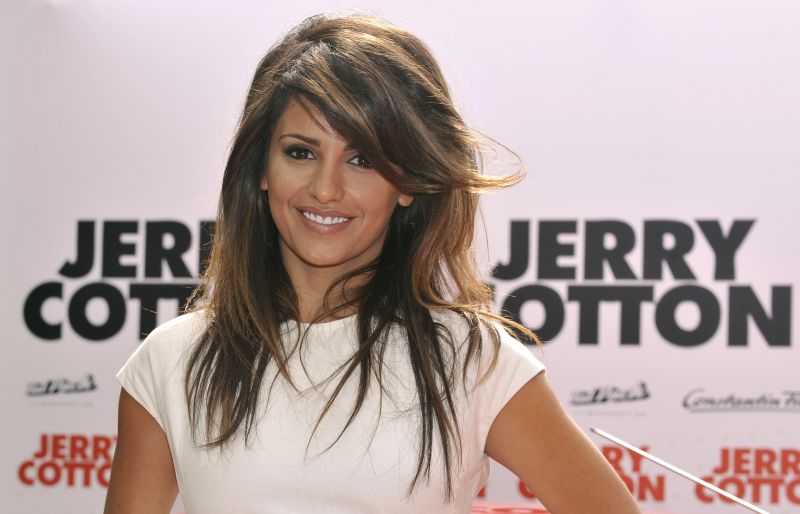This photograph captures a young Penelope Cruz at an outdoor publicity event. She is prominently positioned in front of a billboard adorned with multiple instances of the text "Jerry Cotton." The branding appears in large, all-caps black letters and smaller red letters, consistently repeating across the backdrop. Penelope, displaying her signature vibrant smile, wears a sleeveless white dress. Her voluminous, slightly windswept brown hair partially obscures her face, showcasing the dark makeup applied around her eyes. The background, though primarily obscured by Penelope, features a pale purplish hue accented by repeated brand text, suggesting this is likely a promotional image for the "Jerry Cotton" brand.